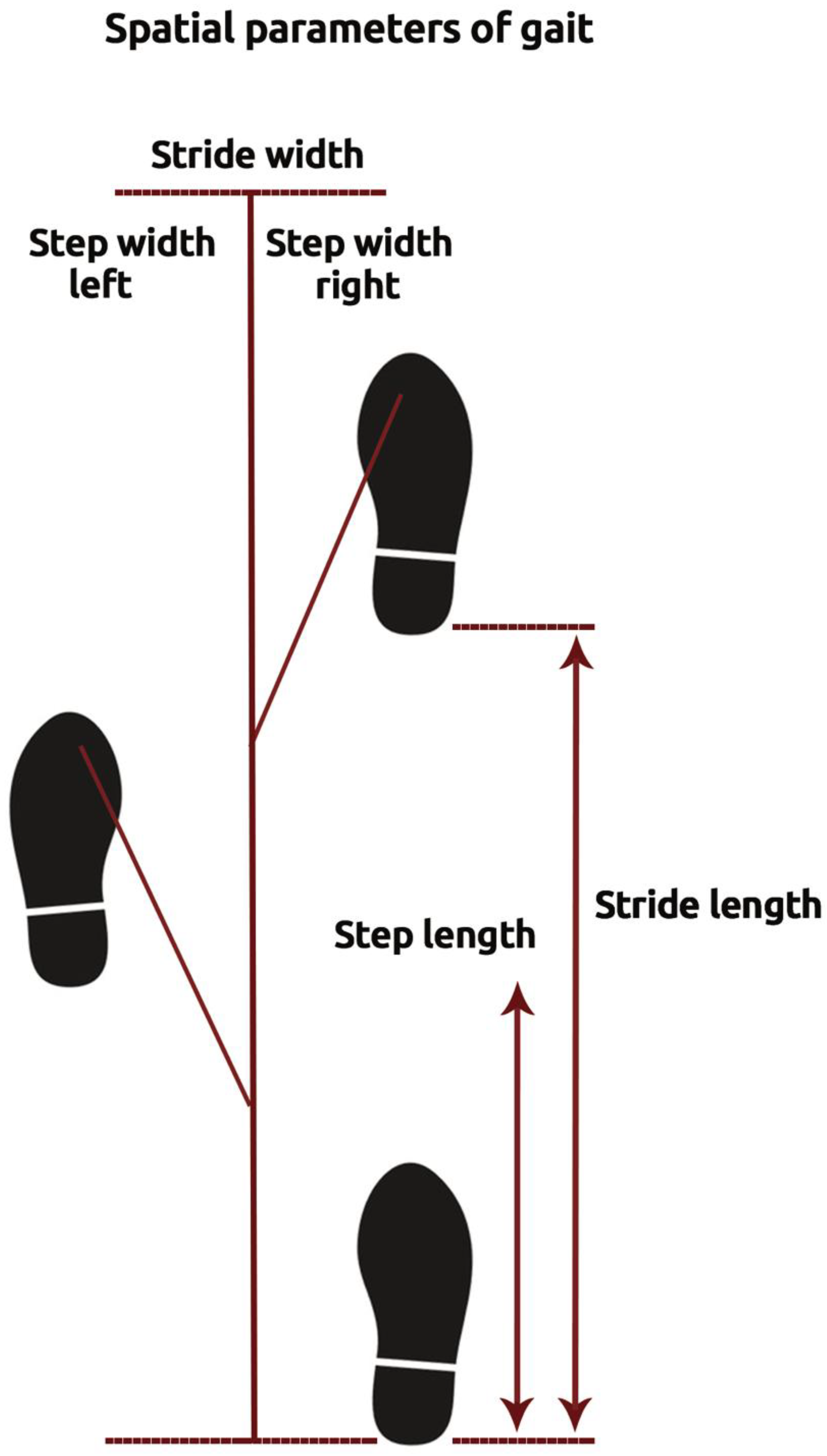This portrait-oriented teaching tool image is titled "Spatial Parameters of Gait" in bold black letters at the top. Below the title, a horizontal red line indicates "Stride Width," and from its center, a vertical red line extends down to the bottom of the image. On the left side of this line, labeled "Step Width Left," is a silhouette of a left shoe sole stemming from the center line. On the right side, labeled "Step Width Right," is a similar silhouette of a right shoe sole. At the bottom of the vertical line, accompanying a horizontal line, is another right shoe silhouette marking the next step. 

The image uses two vertical arrows on the right-hand side for additional parameters: "Step Length," corresponding to the height of the left shoe imprint, and "Stride Length," which measures the distance between the heel of the bottom right shoe imprint and the heel of the next step's right shoe imprint. These details collectively illustrate the concept of gait and its spatial parameters with clear footstep illustrations and labeled measurements.